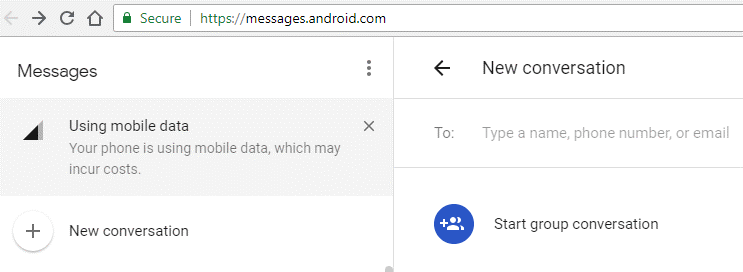Screenshot of the Android Messages app interface (https://messages.android.com). The primary message at the top of the screen notifies the user that their phone is using mobile data, which may incur costs. Below this notification is a tab labeled 'Start chat' situated on the right. The title of the reading pane reads 'New conversation,' and directly underneath is the 'To' field, where one can input the recipient's contact information to initiate a conversation. Adjacent to this is a blue icon for starting a group conversation, understood as part of the text messaging functionality on an Android device.